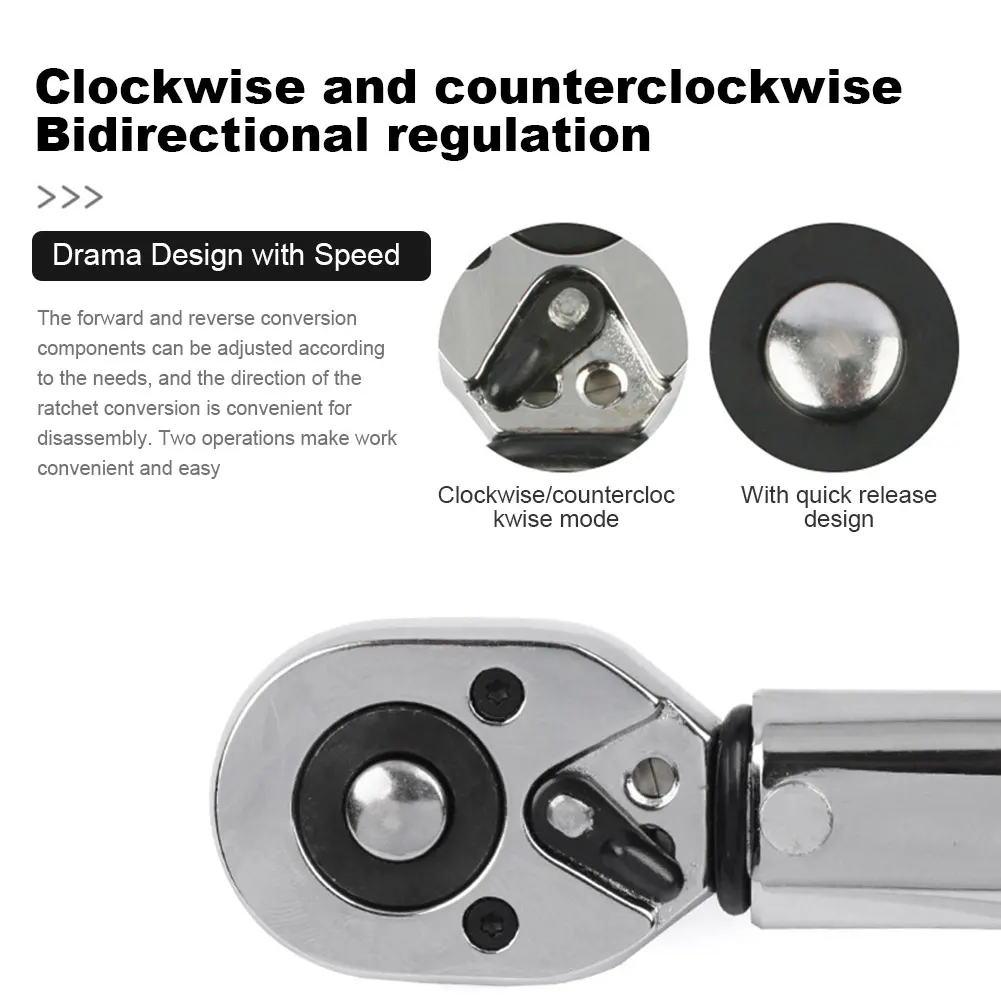The image is an informational piece detailing the features and functions of a ratchet wrench. At the top of the page, in prominent black lettering, it reads "Clockwise and Counterclockwise Bidirectional Regulation." Directly beneath this title, there are three arrows pointing to the right, emphasizing the bidirectional movement. 

Below the arrows, in a black banner with bold white lettering, it says "Drama Design with Speed." Further down, the text describes the "Forward and Reverse Conversion," mentioning that components can be adjusted according to specific needs and that the direction of the ratchet conversion is convenient for disassembly. The description highlights that these two operations make tasks convenient and easy.

To the right of the explanatory text, there are three images showcasing different parts and functionalities of the ratchet wrench. The central image depicts the lever that allows switching between clockwise and counterclockwise modes, marked respectively. Below this is a smaller image labeled "Quick Release," illustrating the quick-release design feature.

Finally, a comprehensive image at the bottom right combines all these elements, showing the full view of the ratchet wrench, highlighting its sleek, silvery chrome color and ergonomic design. The comprehensive view reinforces the product’s convenience, adaptability, and efficiency for various tasks.